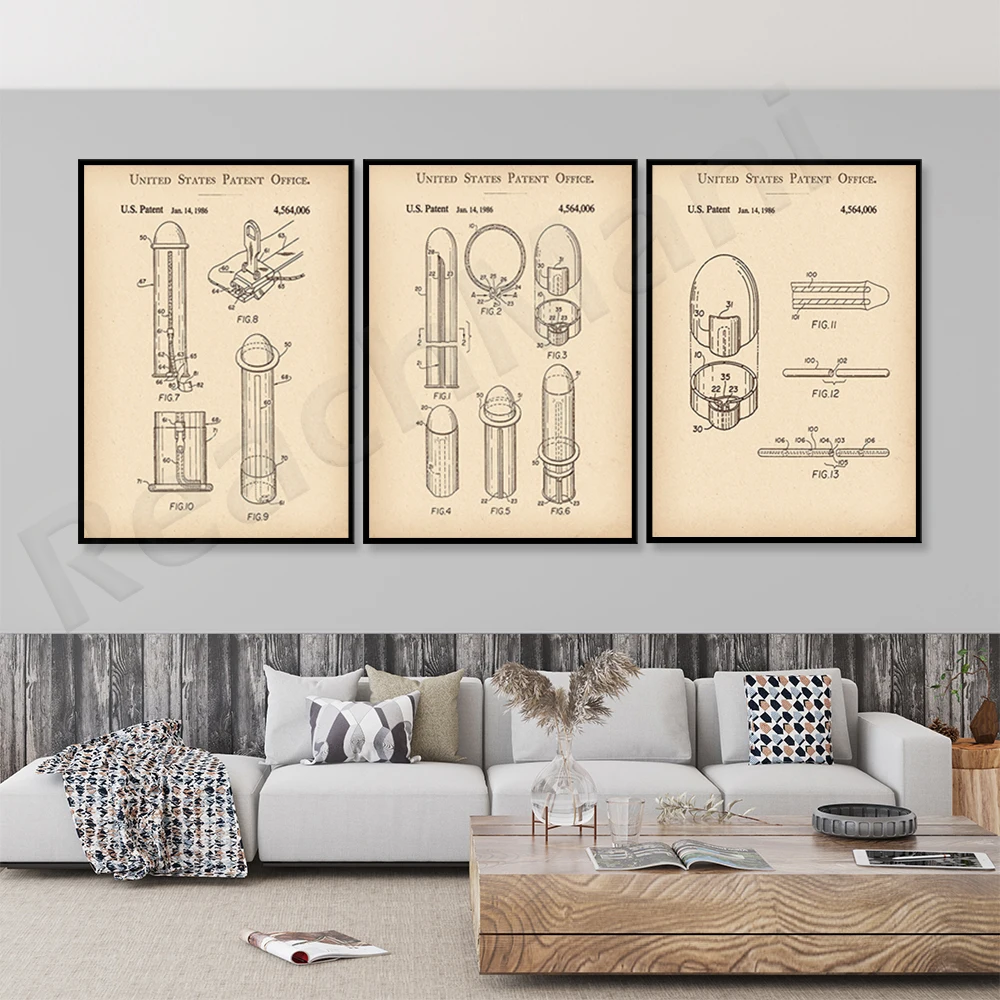The image depicts a stylish arrangement resembling a waiting or living room. Central in the scene is a four-seater, green sofa adorned with a variety of cushions: a gray and white pillow, a couple of gray pillows, a tan pillow, and another pillow displaying a distinctive black, white, and brown pattern. Notably, the leftmost seat of the sofa lacks any back cushions and is complemented by a throw blanket featuring a cross-pattern resting on it. 

In front of the sofa, there is a wooden coffee table composed of two stacked layers. Items on the table include an open magazine, a tablet with a pen on it, a small circular disc with a groove in the center, a clear crystal bowl containing a pen, and several books. Additionally, adjacent to the sofa, there's an ottoman with a matching throw blanket draped over it.

The backdrop wall of the space is characterized by a lower section made of old dried wood planks extending just above the sofa. Directly above this is a plain gray wall. Three large, vintage United States Patent Office posters hang on the gray section, each displaying black and yellow diagrams resembling the dimensions of bullets or other items, adding an intriguing touch to the decor.